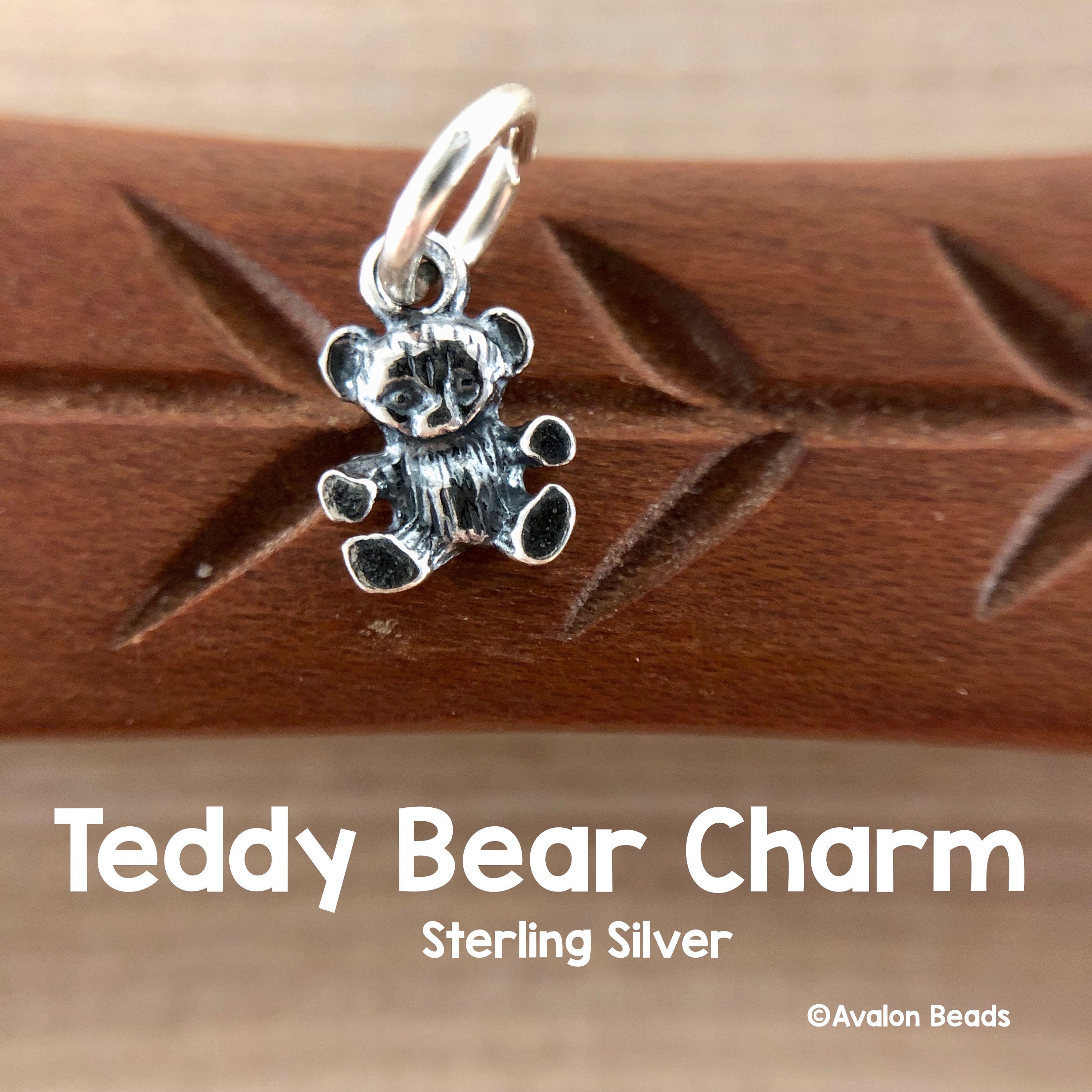The image features a detailed advertisement showcasing a sterling silver teddy bear charm. The charm is prominently centered, slightly towards the upper-left middle of the frame, hanging from a silver or gold hooked loop. It is attached to a horizontally placed engraved piece of wood, which is intricately carved with a design resembling stems with leaf or flower patterns emerging from a horizontal line. The wood's surface and the charm stand out against a blurred wood grain background that adds depth to the image. At the bottom of the picture, "Teddy Bear Charm, Sterling Silver" is written in bold white font, and in the bottom right corner, "© Avalon Beads" is also inscribed in white, anchoring the advertisement with clear brand information.